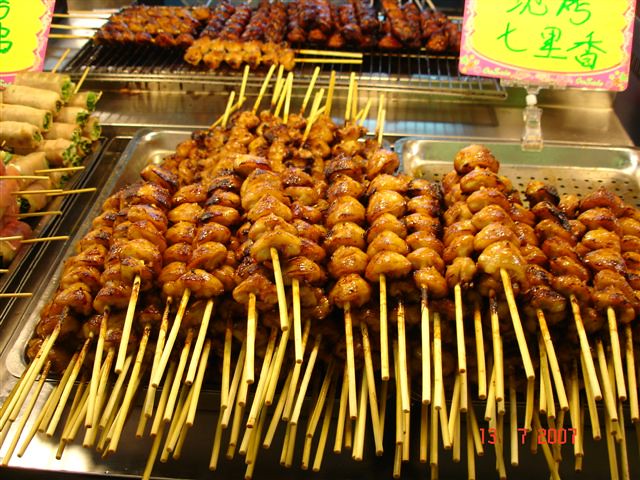In the image, a vibrant food stand in a foreign market showcases an array of tantalizing skewered meats, possibly chicken or other types, neatly arranged on metallic trays. The meat, which appears to be cooked and glazed to a honey-barbecue color, gleams under the lights, highlighting the six round, nugget-like pieces on each skewer. Surrounding the food stand are signs with Asian writing, signaling this could be an Asian market, though the text is unreadable. In the foreground is a silver tray brimming with skewers, each meticulously organized, and a pile of extra sticks lies nearby. In the background, additional trays display a variety of other skewers. Notably, to the left of the main tray, there are rolls that could be egg rolls or spring rolls, wrapped in dough and hinting at a broader selection of delicacies available at this enticing food market. The scene is set on a metal countertop, with a pink card featuring green text and a number sequence at the bottom right: 13, 7, 20, 13, 7, 2007.